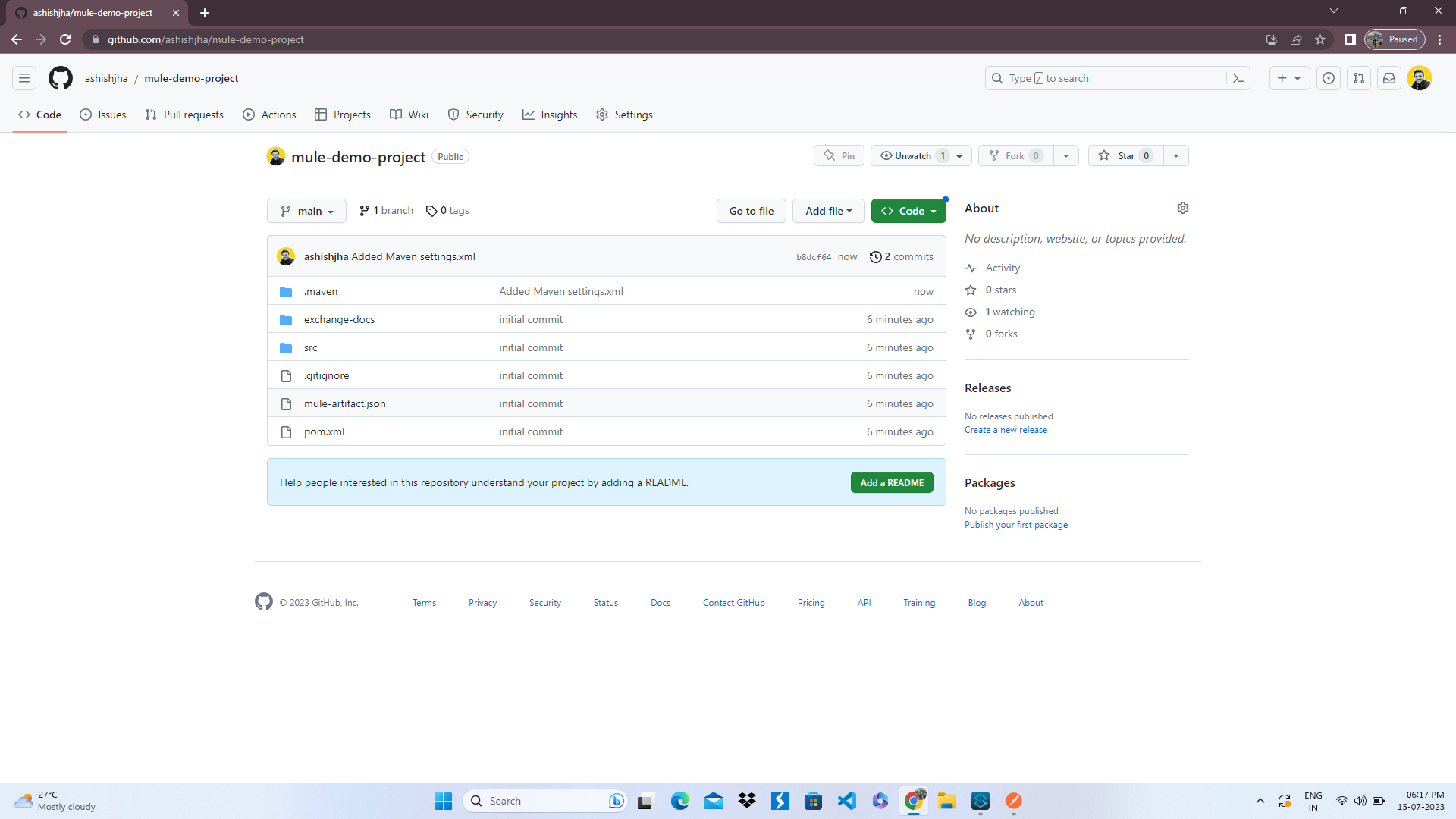A detailed screenshot of a browser page is shown. At the very top, a black banner is present with a search bar embedded within it. This banner also houses a back button and a forward button on the left, depicted as arrow icons, and a refresh button to the right of the forward icon. 

The browser tab is open, displaying minuscule white text, suggesting that the screenshot might have been minimized. Below the black banner, the page itself has a gray background. At the top of this, a very small username or filename and a logo are visible.

Just beneath, there is a navigation panel with various options including "Code," "Pull requests," "Projects," "Wiki," "Security," "Insights," and "Settings." Following this panel, the main content area of the page features a large, white background. Centrally positioned within this background is a prominent square panel that reads "Multi Mule Demo Project." There is an edit button next to this title that allows for editing.

The page contains multiple selections and file names with their respective upload dates listed below the central panel. Towards the lower section, a blue bar spans the width of the content area and includes a prompt to "Add a README" on the far right side.

The bottom portion of the screenshot reveals the person's desktop taskbar. This includes various icons, a search bar, and, on the far right, indicators for the time and Wi-Fi signal.